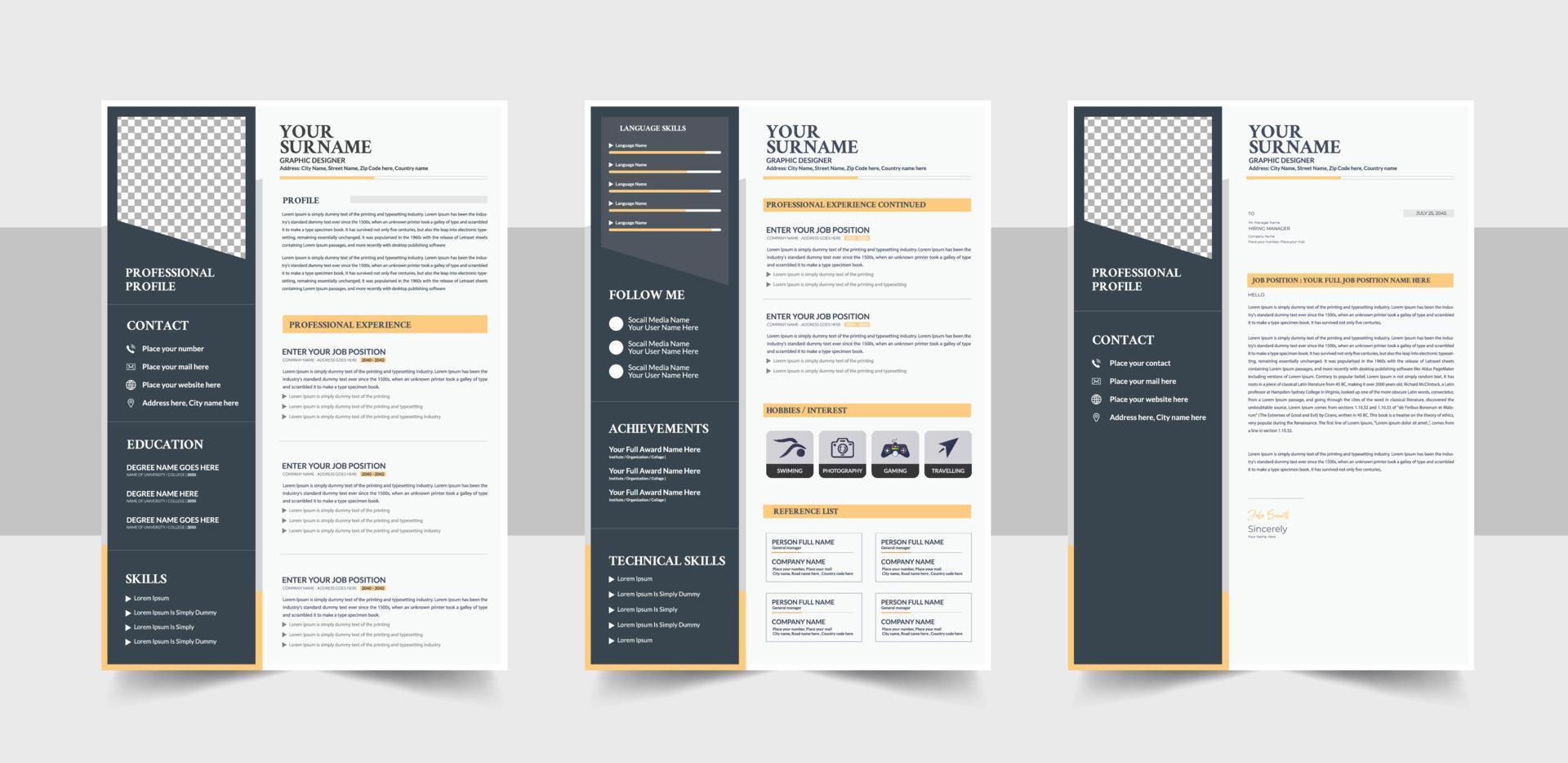The image showcases three detailed resume templates, each designed to assist in the creation of a professional profile. At the top of every template, there's a placeholder marked "Your Surname," indicating where one's name should be entered. 

The first template emphasizes a professional profile section, accompanied by a sidebar on the left listing contact information, education, and skills. This layout is characterized by black text and gold highlights.

The second template also begins with "Your Surname" at the top and includes sections for a professional profile, contact information, follow-me links, achievements, and technical skills. Notably, the layout divides the page into thirds, with the left third featuring a darker color, possibly black, while the right side contains the main text.

The third template features a professional profile, contact information, education, and skills sections, similar to the first but with a different arrangement of text lines where the information is to be filled in. All three templates share a cohesive black-and-white color scheme with gold accents, set against light and dark gray backgrounds, making them both professional and visually distinctive.